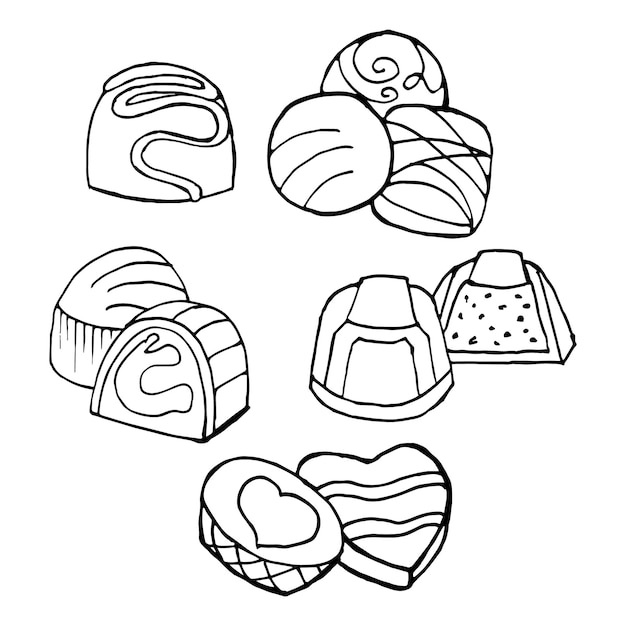The image features detailed black and white digital drawings of various chocolates set against a solid white background. At the bottom middle, there are two prominent chocolates: one circular piece decorated with a heart design and a lattice-style crisscross; next to it, a heart-shaped candy with two wavy horizontal stripes. In the top left corner, there is a singular chocolate resembling a round piece of bread with a distinctive S-shaped squiggle on it. Scattered around these are additional pieces of chocolates, with some placed in the top right corner and the upper left vicinity, varying in shapes including round, oval, and heart-shaped, and adorned with intricate patterns. Some chocolates appear bitten, revealing their inner fillings, enhancing the authenticity and charm of the drawing.